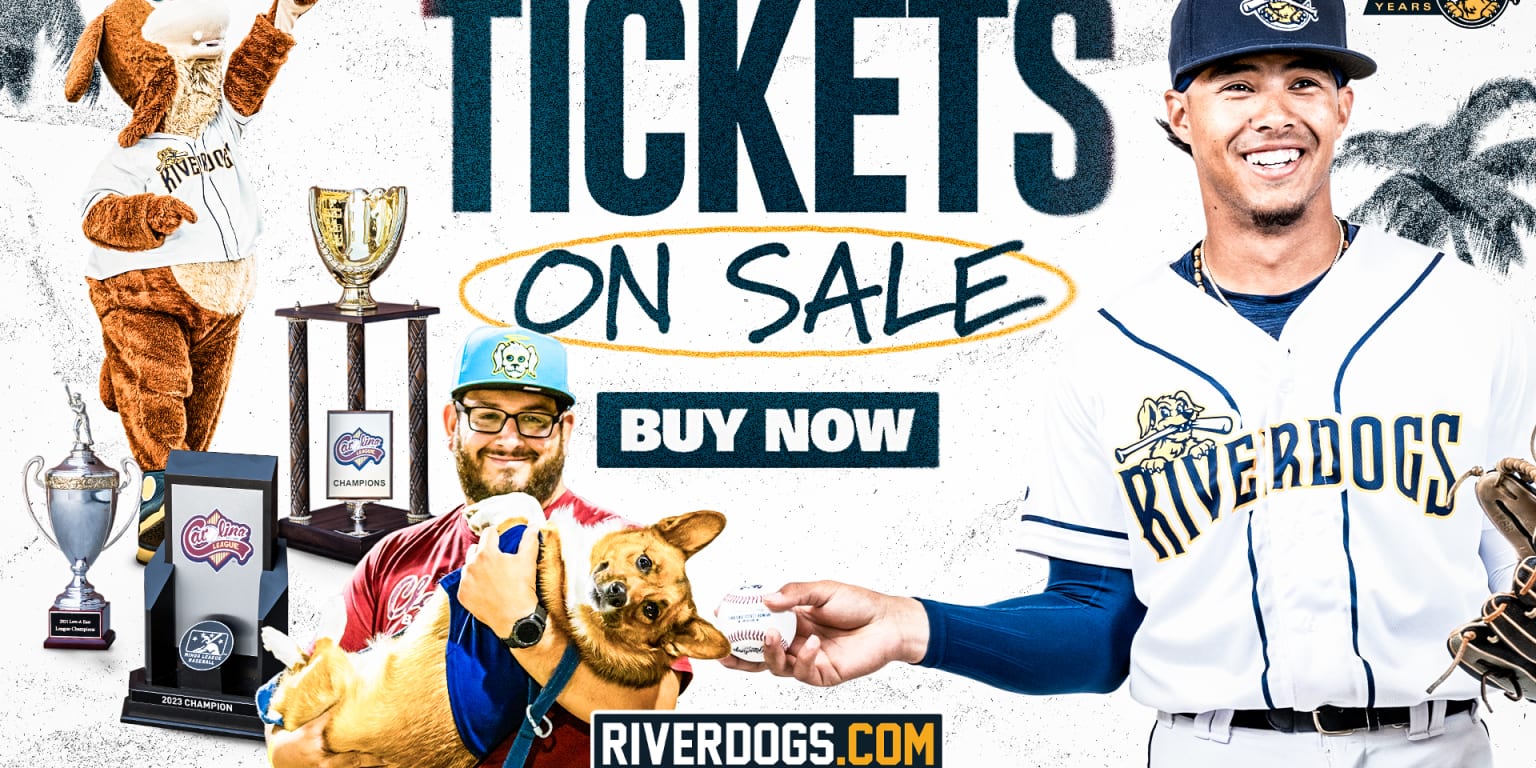The image is an advertisement, possibly on a website, featuring a promotional banner for the Riverdogs baseball team. At the top of the ad, in large, dark navy blue, all-caps letters, it says "TICKETS." Below this, in a handwritten-style, all-caps font circled with yellow, it says "ON SALE." Further down, in white letters against a blue rectangular background, it says "BUY NOW." At the bottom of the image, the website "RIVERDOGS.COM" is prominently displayed in all caps.

To the right of the text, there is a young man dressed in a white baseball uniform with blue stripes, wearing a navy blue cap and a white shirt with the team name "Riverdogs" emblazoned across the front. He holds a baseball in his outstretched right hand and wears a glove on his left.

On the left side of the image, there are several trophies indicating the team's achievements. Above the trophies, partially overlapping them is a mascot wearing a brown costume and a white shirt with "Riverdogs" on it. Additionally, there is another man with a beard and glasses wearing a light blue cap, holding two dogs in front of him. The overall background of the ad is white, giving prominence to the text and images.